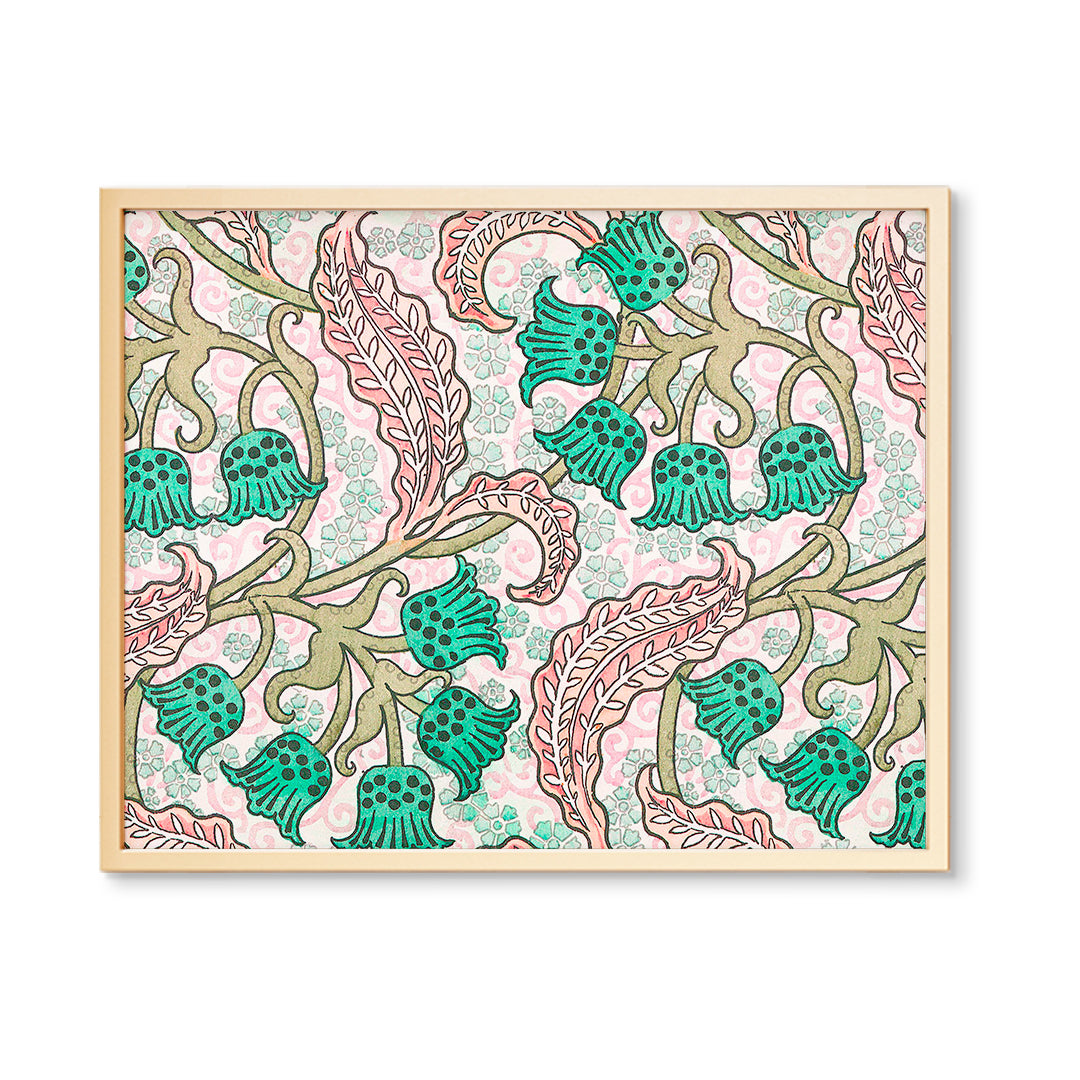This illustration is housed within a thin, light brown frame which may be metal, although that's uncertain due to the shine on its right side. The background is predominantly light pink, setting the stage for an intricate botanical design. At the heart of the artwork are green blossoms shaped like bells, sporting dark green to bluish dots and lines that climb up their petals. These flowers are clustered atop twisting stems of varying hues from yellowish-green to brown. Surrounding these are large, pastel pink leaves with curly points and detailed, fern-like inner patterns.

Interspersed throughout the background are faint but noticeable lighter blue flowers and delicate clovers, enhancing the layered composition. Brown vines wind through the scene, adding a touch of contrast and complementing the overall muted color palette, save for the vibrant blue-green blossoms. This meticulous arrangement of flowers and leaves suggests a whimsical yet structured aesthetic, blending natural elements with abstract design.